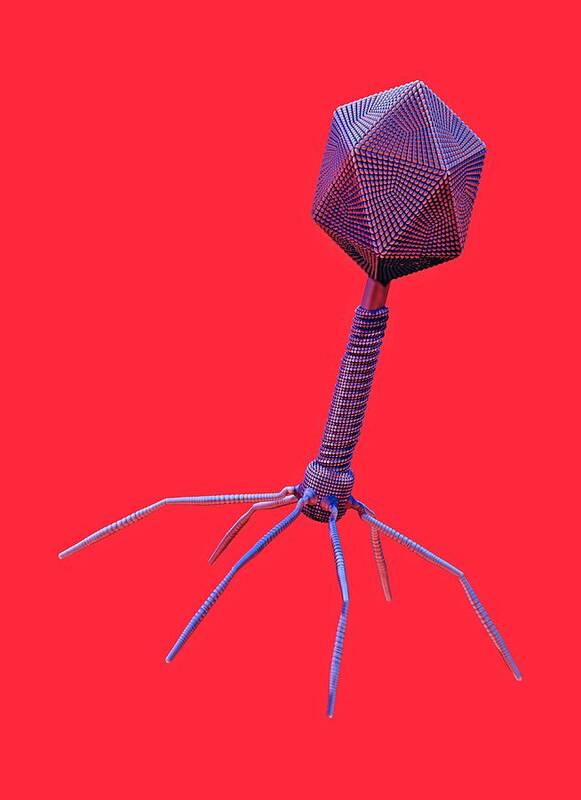This image is a highly detailed and dramatic computer illustration, featuring a microbial- or virus-like structure set against a striking red and orange background. The main object is predominantly silver and purple, characterized by a top section that showcases an intricate geometric shape with numerous facets, resembling a decahedron. The structure continues down into a slender tube-like neck that connects to a larger, more robust cylindrical section adorned with a squarish, segmented pattern. This cylinder has six spider-like, multi-segmented legs radiating outwards, giving the object an almost futuristic and robotic insect appearance. The object is angled slightly to the right, with some legs potentially lifted off the ground, enhancing its dynamic and eerie presence against the vivid backdrop.